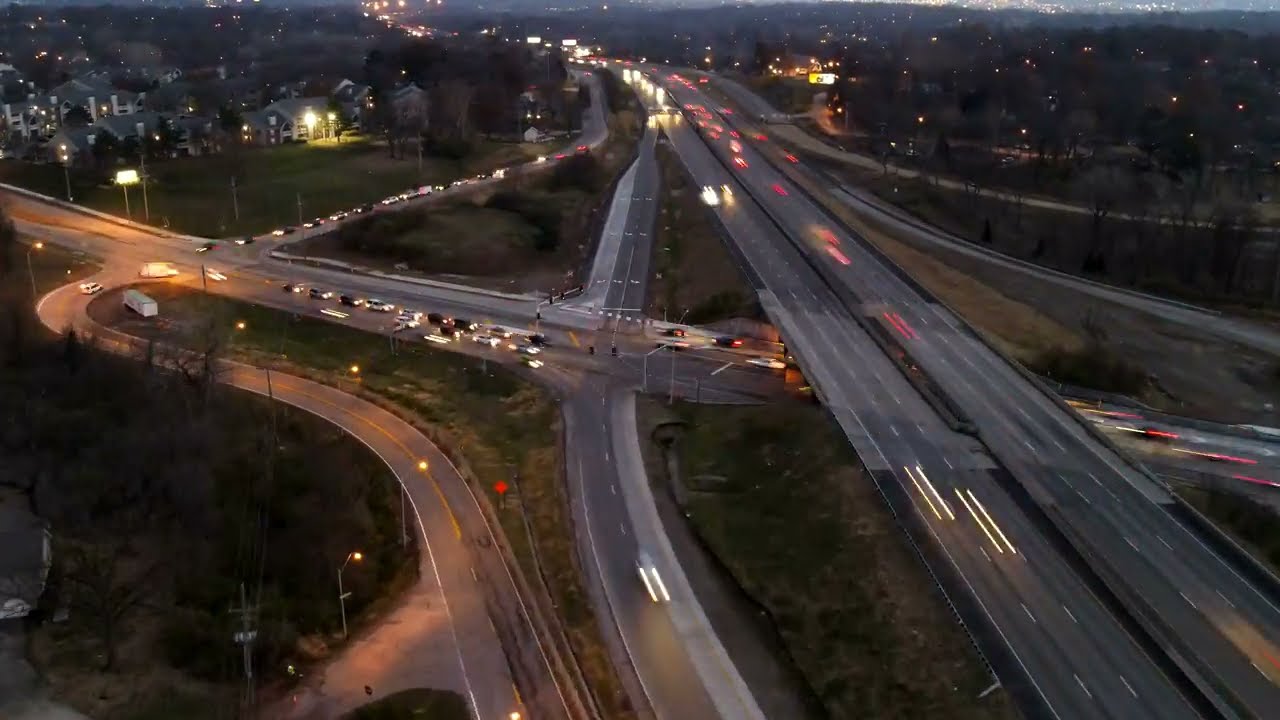This image captures an intricate freeway system near a small metropolitan area, likely at dusk or early night. The primary scene features two major highways crisscrossing each other, with multiple on-ramps and off-ramps weaving off in various directions. One prominent highway runs from the bottom to the top of the image and is intersected by another large interstate type road stretching from left to right. A secondary road curls from the top middle, looping around and connecting with the main highways. Although the region is predominantly paved, there are sparse patches of grass visible, along with numerous streetlights illuminating the scene. Scattered cars with headlights and brake lights indicate light traffic on these expansive roadways. In the background on both the left and right sides, suburban characteristics emerge with apartments, residences, and smaller buildings, their lights glowing softly against the darkening sky.